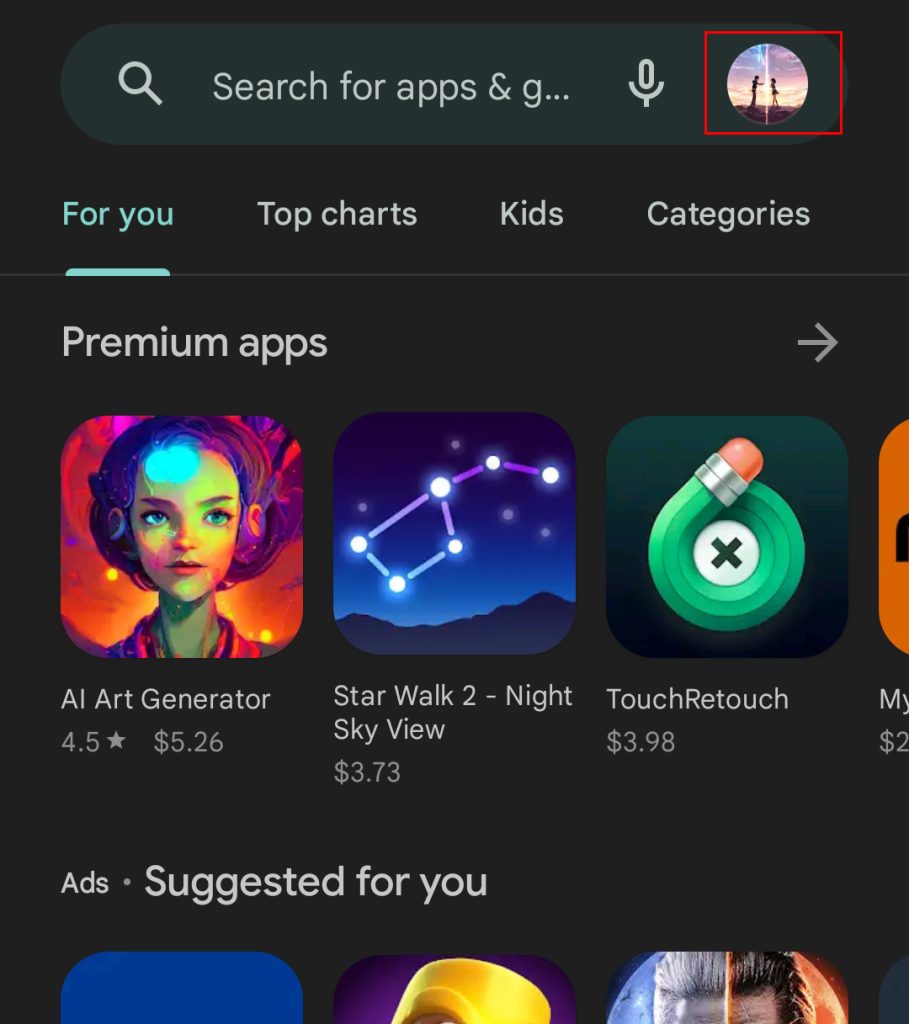The image is a screenshot of a digital storefront with a gray gradient background transitioning from black at the top to lighter gray at the bottom. At the top of the screen, there is a prominent search bar accompanied by a magnifying glass icon, with the prompt "Search for apps and games..." partially visible, indicated by "G...". Beside the search bar, there are icons for a microphone and circular avatars, suggesting voice search and user profile options respectively. The user's profile picture is highlighted with a red rectangle.

Directly below the search bar, there are segmented tabs labeled "For You" in green, "Top Charts," "Kids," "Categories," "Premium Apps," and a navigation arrow pointing to the right. Following these tabs, the first app listing is an "AI Art Generator," rated 4.5 stars and priced at $5.26. Next is "Star Walk 2: Night Sky View," priced at $3.73, followed by "Touch Me Touch," priced at $3.98 and indicated to include ads.

Further down, there is a section titled "Suggested for You," which is partially cut off. Within this section are three app icons arranged in a horizontal row: the first icon is blue, the second is purple with a yellow object in the middle, and the third is red on the right and blue on the left, featuring the image of a man.